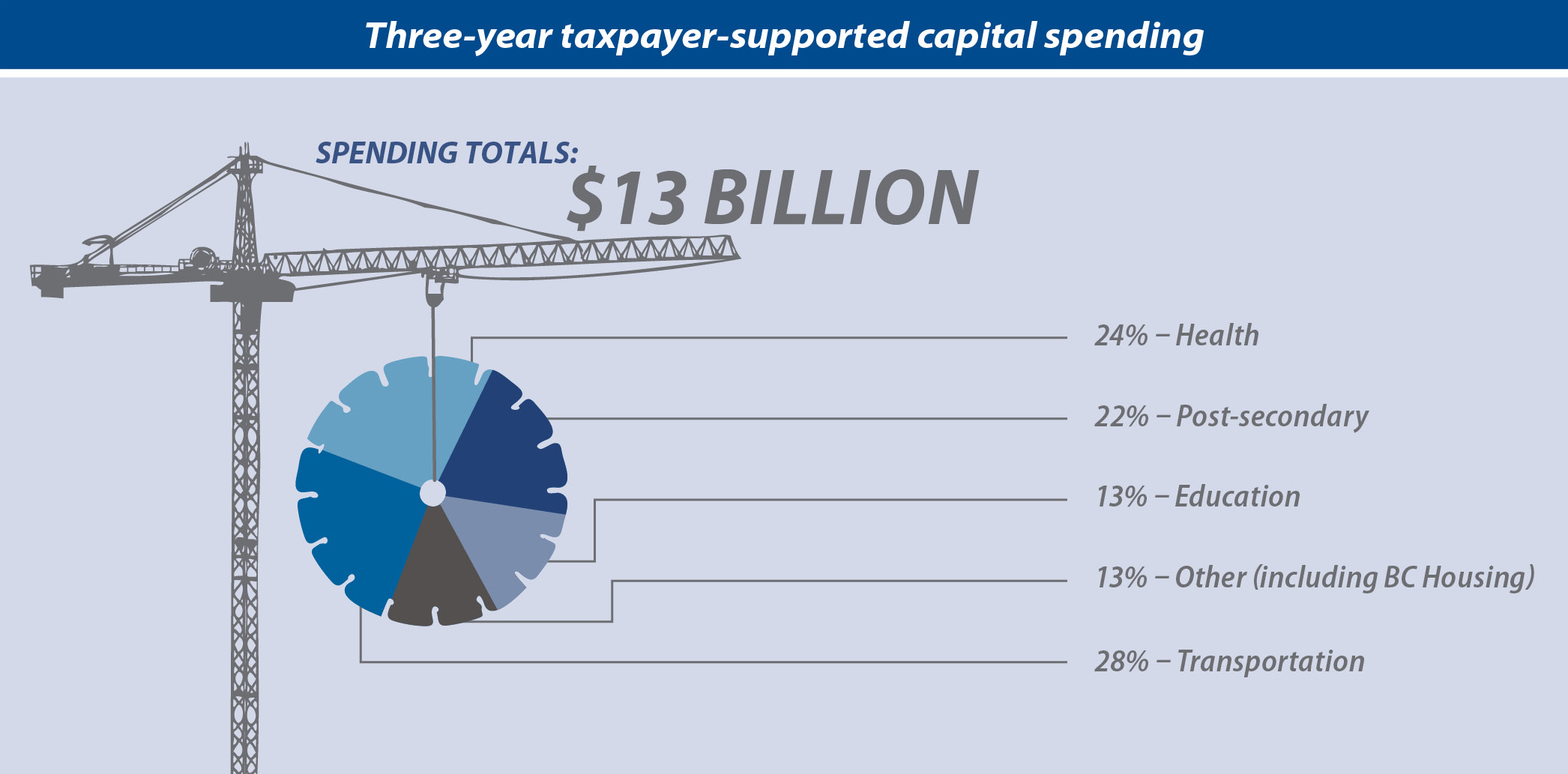The image is an infographic that appears to be from a presentation, showcasing three-year taxpayer-supported capital spending. Dominating the visual is a tall, gray silhouette of a sky crane on the left-hand side, with its arm extended downwards. Hanging from the crane is a cleverly designed pie chart that resembles a large, saw-like wheel. This pie chart is segmented into different colors, including shades of blues and grays, each representing a portion of the spending allocations.

At the top of the image, a navy blue band stretches horizontally with the text "Three-Year Taxpayer-Supported Capital Spending" written in bold white font. Just below this, the background transitions into a light gray-blue.

Positioned centrally beneath these elements, the infographic states "Spending Totals: $13 billion" in gray text. The pie chart is divided into five sections, each connected with lines to corresponding percentage breakdowns listed in gray text. These sections indicate that 28% of spending is allocated to transportation, 24% to health, 22% to post-secondary education, 13% to education, and another 13% to other areas, including BC housing. The overall color scheme features blue and gray tones, providing a clean and visually appealing representation of the data.